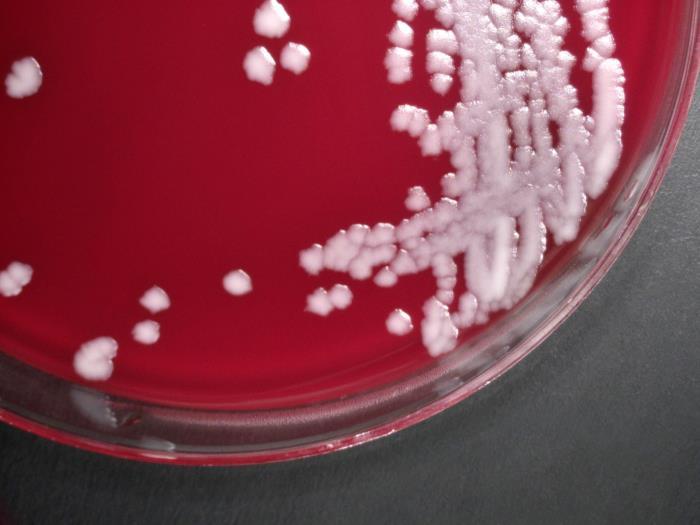The image depicts a zoomed-in, vertically-standing, thin circular glass container, reminiscent of a Petri dish. The container features a solid red bottom and contains a cloudy white liquid with various white droplets dispersed throughout. The droplets are clustered mostly on the right side of the container, gradually separating towards the left. The container rests on a gray, stone-like surface, and a white reflection is visible on the bottom right of the glass. The overall image has a slightly blurred quality, with no text or additional description to provide further context.